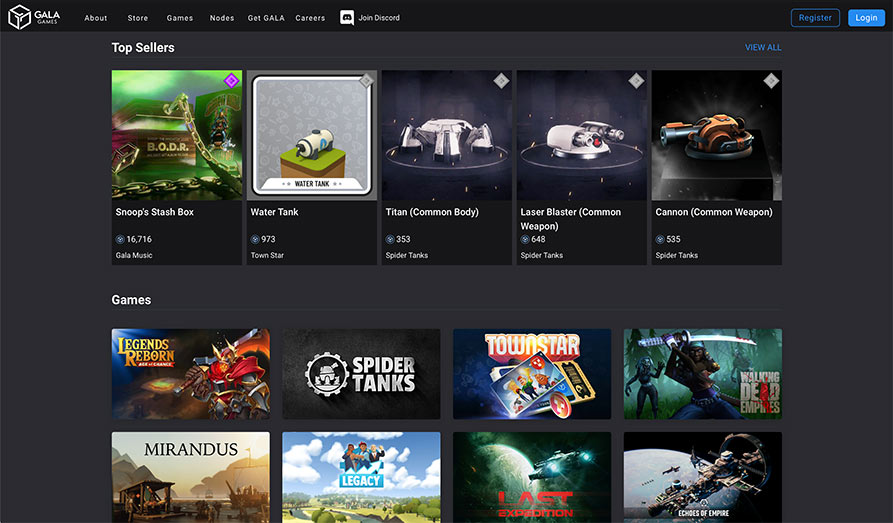The image depicts a digitally rendered interface with various elements arranged systematically from top to bottom. At the top, there is a prominent black line. Adjacent to this, there is a white-outlined square with the word "GALA" next to it, possibly a logo or a title. Below this, there is a series of smaller, illegible words, arranged in a sequence. Alongside this sequence, there is another white square with an indistinct symbol or content inside it, accompanied by a word that is too small to discern.

Moving towards the right, there is a blue-outlined rectangle containing an inscrutable blue word. Next to it, a solid blue rectangle bears the word "LOGIN" in white font. Following this, a lighter gray rectangle is visible. The top section of this gray rectangle is labeled "TOP SELLERS," and beneath this heading, there are various icons that appear to represent different games, marked by small titles in black rectangles with writing too small to read.

Further down, the section labeled "GAMES" displays a collection of eight game thumbnails. Despite the small size of the text, one game title, "SPIDER TANKS," is legible among the listed games. There are also five movies depicted within this interface, though the specific details on these remain indistinguishable due to small text size.